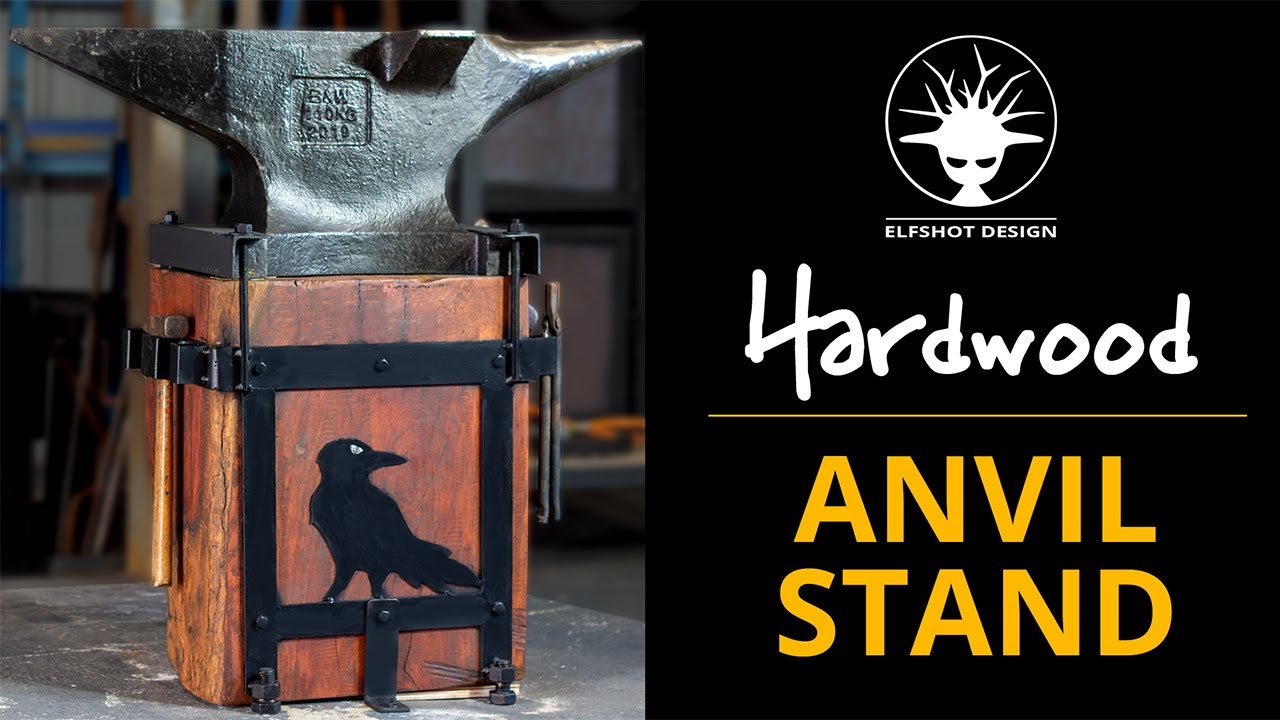The promotional image features a meticulously crafted black cast iron anvil mounted on a hefty brown wooden block. This wooden block is reinforced with a black metal frame that displays a stylized metal outline of a crow on one of its faces. The left half of the image prominently showcases the anvil setup. The right side has a black border adorned with various inscriptions. At the very top of this border, a white circular logo depicts an elf-like figure with branch-like protrusions growing from its head, giving it a somewhat eerie appearance. Directly beneath the logo, the text in white reads "Elf Shot Design," indicating the company behind the product. Below this, the word "Hardwood" is displayed followed by a thin yellow line and the text "Anvil Stand" in yellow, completing the branding and product name.